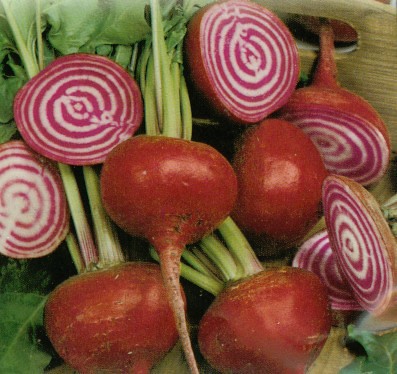This detailed photograph captures a close-up of several Guardsmark beets nestled within a wooden crate. The beets, characterized by their vibrant red exterior, are presented both whole and sliced to reveal their stunning interior pattern. Sliced sections showcase the beets' distinctive concentric circles of alternating deep red and dark red-pinkish swirls, reminiscent of a peppermint swirl or an archery target. The green stalks emerging from the beets add a contrasting burst of color and are prominently displayed at various points around the image. The setting appears rustic, suggested by the visibility of a hand hole in the wooden crate behind the beets, adding to the earthy charm of the scene.